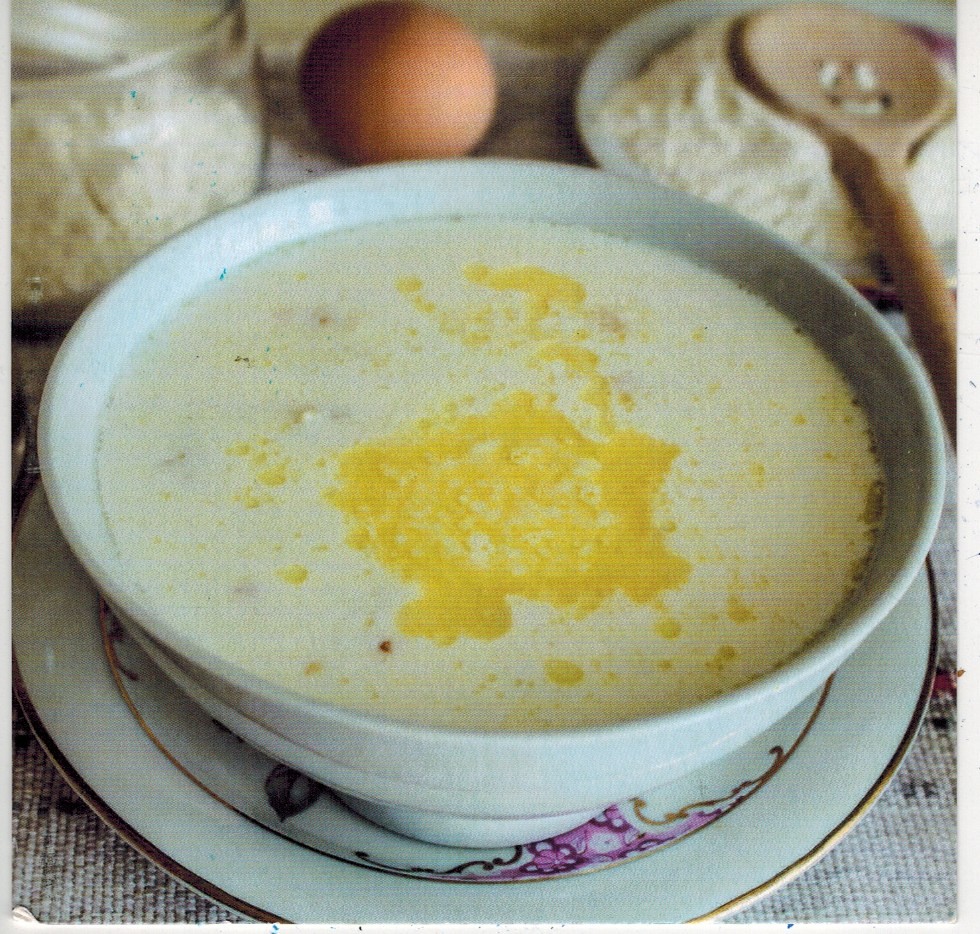The photograph showcases a white porcelain bowl filled with a creamy, white liquid, almost to the brim, with small yellow drizzles and tiny bubbles concentrated towards the center, likely from melted butter or oils. This bowl is situated on a matching white plate that features an elegant gold trim and various purple floral designs, including a gold circle around its inner rim. Both the bowl and plate rest on a table adorned with a burlap sack-like tablecloth of a whitish-brown hue. In the background, slightly blurred, there is a single brown chicken egg placed next to another white plate covered in flour. A wooden spoon rests on this flour-covered plate, adding a rustic touch. The background also includes a glass container filled with more flour, creating a quaint, homey kitchen scene.